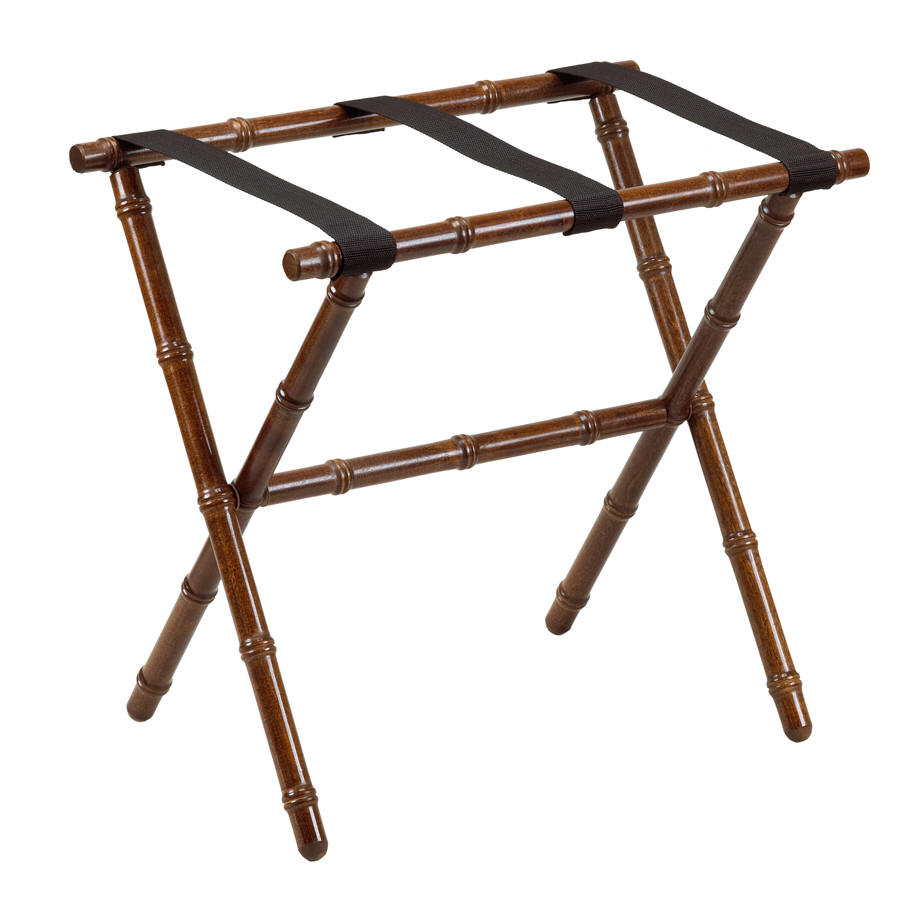The image features a wooden object set against a pristine white background, emphasizing its three-dimensional appearance. Crafted from dark-stained wood with characteristics similar to bamboo, the piece showcases four crisscrossing legs that form an X-shape when viewed from the side, providing stability and functionality. Each leg is adorned with subtle markings reminiscent of bamboo's natural joints, enhancing its visual appeal. The top section of the object is equipped with three black elastic bands stretching across the open area. This design suggests it is a specialized piece of restaurant equipment, likely used by waiters to hold multiple serving trays or dishes, facilitating efficient table service in busy dining settings.